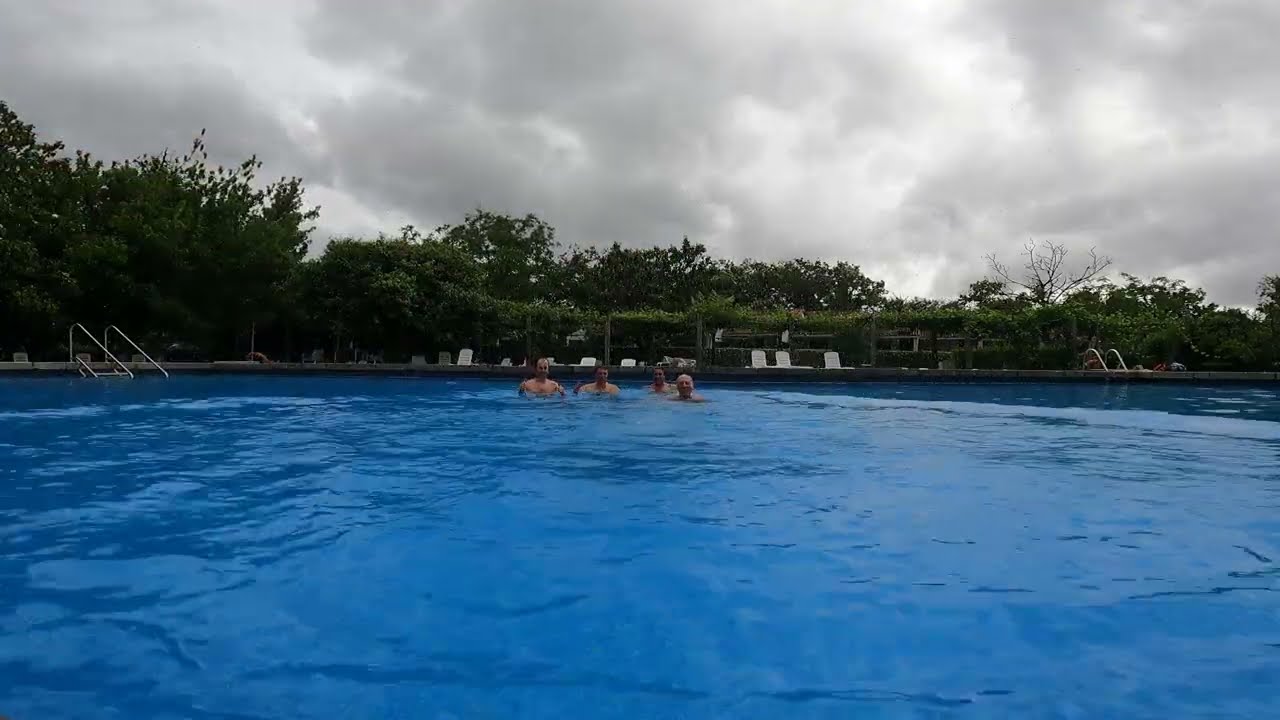This photograph captures an expansive, beautiful blue swimming pool, occupying the entire bottom half of the landscape-oriented frame. The water, which is a dark, clear shade of blue, appears serene and inviting despite the overcast weather. At the midline of the image, four men are seen submerged up to their shoulders, posing towards the camera. The background features several white pool chairs and two silver handrails for pool entry, enhancing the impression of a public pool with ample seating and access points. Behind the pool area, lush green trees and foliage provide a natural border. The upper third of the photograph is dominated by a dark, dreary sky filled with grayish-black clouds that hint at an impending storm, adding a dramatic contrast to the otherwise tranquil scene.